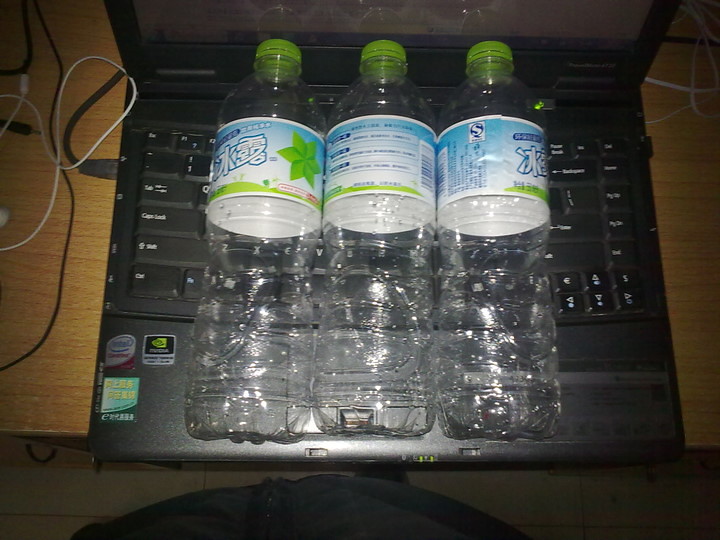The image captures a detailed scene of a tabletop with a wood grain design. At the bottom of the photo, part of the photographer's shirt is visible, including a black zipper and possibly a black shoe or sock. The table features a white tile floor beneath it. Central to the image is a black laptop, which is open and appears to be displaying a web page. The laptop has several stickers, including one that reads "Intel," and features black keys with white writing. Surrounding the laptop are an assortment of wires—two black cords and one white, potentially for headphones. On the laptop's keyboard lie three empty, clear plastic 20-ounce bottles. Each bottle has a lime green cap and a label with blue, white, and green colors, featuring some sort of Asian script, possibly Chinese or Japanese, and a star-like green design.